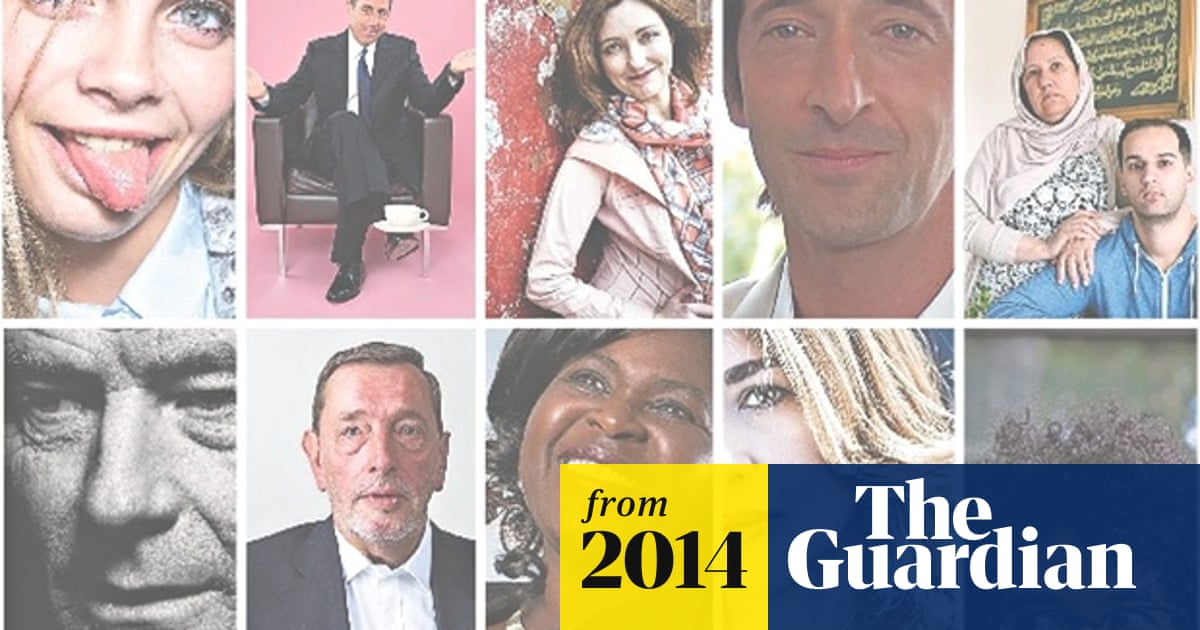The image is an advertisement for The Guardian from 2014, featuring a grid of 10 photographs of people arranged in two rows, with five pictures on the top row and four on the bottom row. A superimposed banner with a yellow section stating "from 2014" in black block letters, and a navy blue section with "The Guardian" in white block letters spans across the last three pictures on the bottom row.

In the top row, starting from the left:
1. A woman sticks out her tongue.
2. A man in a business suit sits in a chair.
3. A woman stands against a wall in a pink dress with a plaid scarf, with short brown hair.
4. A close-up of a man with short brown hair wearing a white shirt.
5. A man in a cyan colored jacket with short brown hair is seated with a woman in a burqa leaning on him.

In the bottom row, starting from the left:
1. A black and white close-up of an old man’s face.
2. A man in a tuxedo with short brown hair.
3. An African American woman with short brown hair, partially cut off by the banner.
4. A woman’s face partially cut off by the banner, showing blonde hair and brown eyes.
5. An individual with curly hair not visible due to the banner.